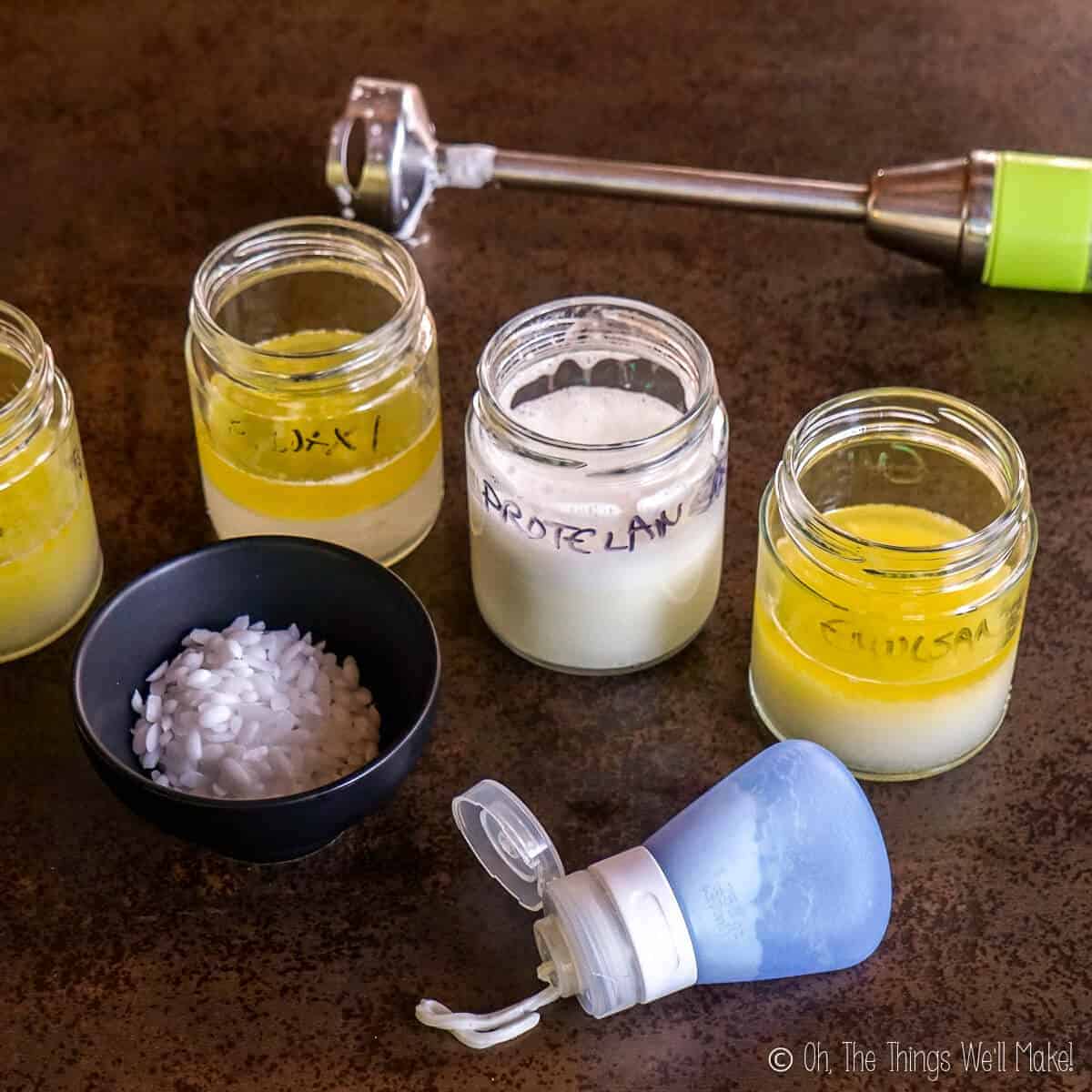The photograph features a collection of four small jars, each approximately three-quarters filled with various substances, likely intended for some form of creation or crafting. The jars are arranged on a brown, grainy surface that resembles a kitchen countertop. In the bottom right corner of the image, the text "© Oh, the things we'll make" is written in white letters, suggesting a theme of creativity and experimentation.

From left to right, the jars contain different materials. The second jar is labeled "WAX," indicating it's filled with melted wax. Next to it is a white jar labeled "PROTELAN," which might contain some form of protein or thickening agent. The far-right jar's label is obscured and unreadable. A small, dark bowl filled with grains or a grainy substance is positioned in front of the second jar from the left. Nearby, there's a shaker that resembles a pepper shaker and a handheld immersion blender, hinting at the mixing and preparation of the substances in the jars. The visually rich display evokes a sense of curiosity and inventiveness.